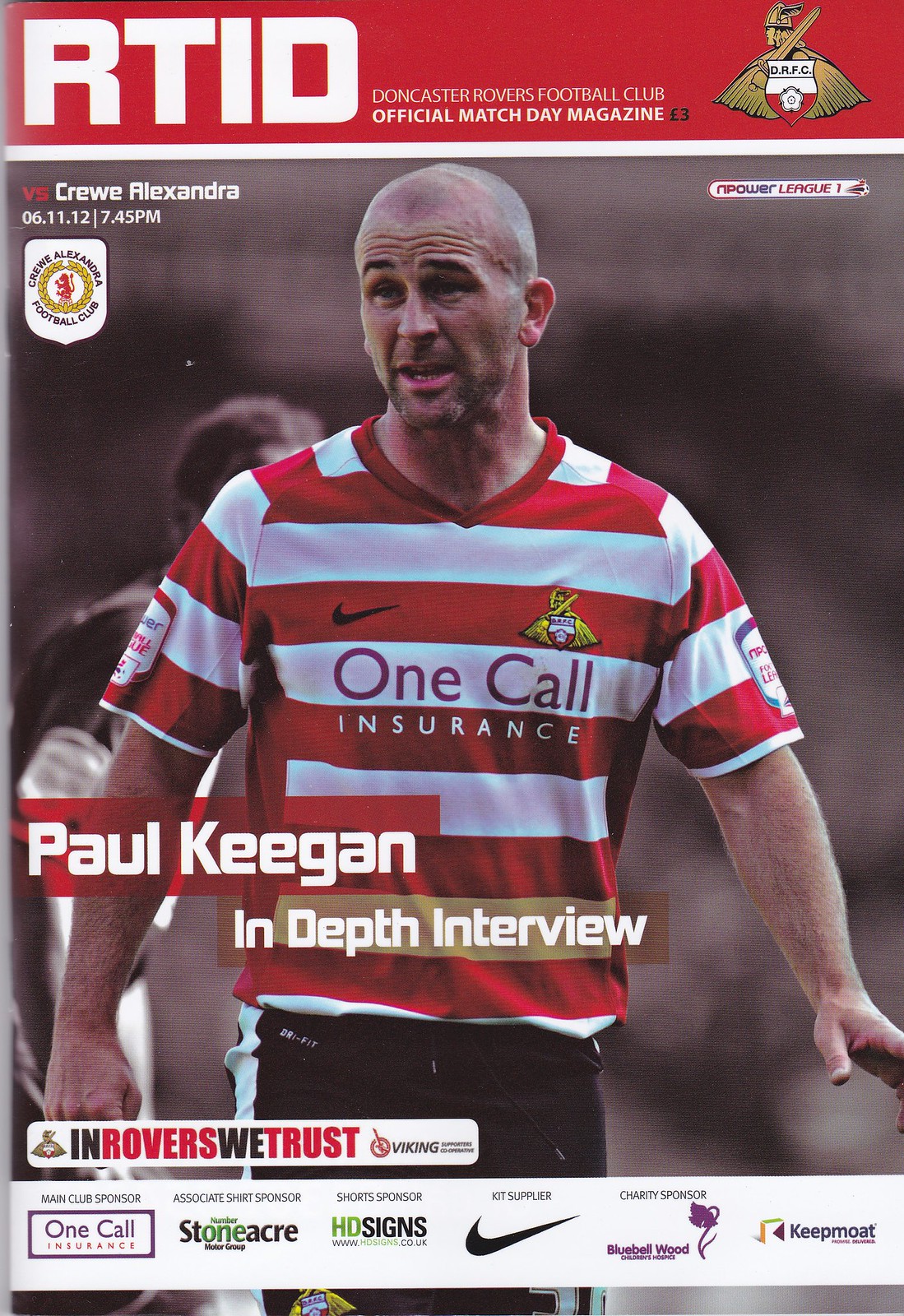The cover of the official matchday magazine for Doncaster Rovers Football Club, titled "R.T.I.D. Doncaster Rovers Football Club Official Match Day Magazine," is prominently featured. The top section has a red bar with white text indicating the magazine's title, priced at three pounds, and includes the club's Viking-themed crest adorned with a Nike swoosh in gold. To the right of the title are details about the match against Crewe Alexandra, scheduled for November 6, 2012, at 7:45 PM. The main image centers on footballer Paul Keegan, who is identified by overlaid white text announcing an "in-depth interview" with him. He wears a red and white horizontally striped jersey sponsored by OneCall Insurance, and black shorts, as he walks on the field. Below the image, the slogan "In Rovers We Trust" appears, accompanied by logos of various sponsors, including Nike, Stoneacre, HD Signs, Keepmoat, and OneCall Insurance.